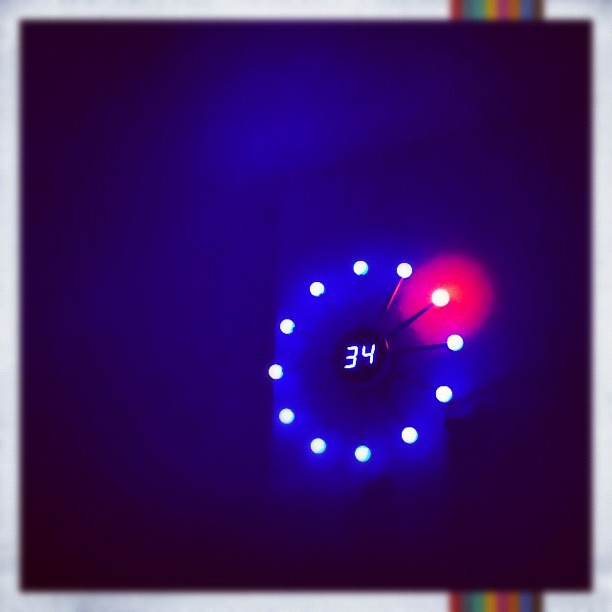This image captures a dimly lit scene dominated by a glowing wall clock. The surrounding background is a deep, dark blue hue, accentuated by a highlighted, round, pink area on the wall, which provides a subtle focal contrast. The clock itself features illuminated white circles, brightly marking the positions where the numbers 1 through 12 would typically reside. Uniquely, the number "34" is conspicuously centered on the clock face. Radiating from the clock's center, sharp spikes extend outward, marking the hours in place of traditional numbers. The overall image has a slight blur, adding a dreamy, ethereal quality to the glowing elements.